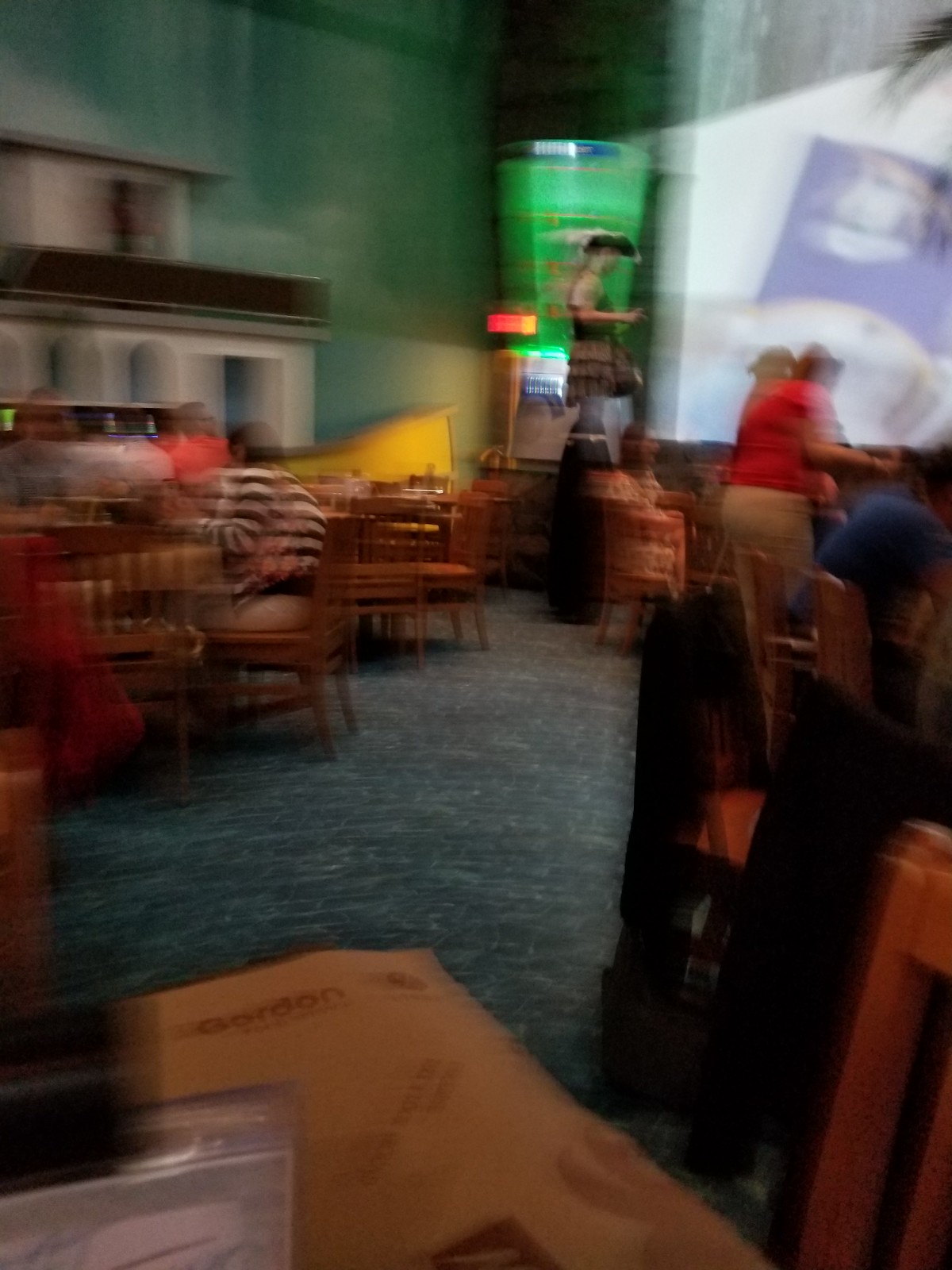The photograph depicts the interior of a restaurant or café with a somewhat blurred focus, making the finer details slightly challenging to discern. Dominating the right side of the image is a projected display or a white screen affixed to one of the walls, glowing with an unclear image. In front of this screen stands a person clad in a bright red shirt, whose shadow is cast prominently against the illuminated backdrop. The venue features numerous wooden tables and matching chairs that accentuate a warm, inviting ambiance. Adding a pop of color to the oak furnishings, the floor is adorned with a deep blue carpet. Despite the blurriness, a few patrons can be seen seated at the tables, engaging in quiet conversations, contributing to the laid-back atmosphere of this dining space.